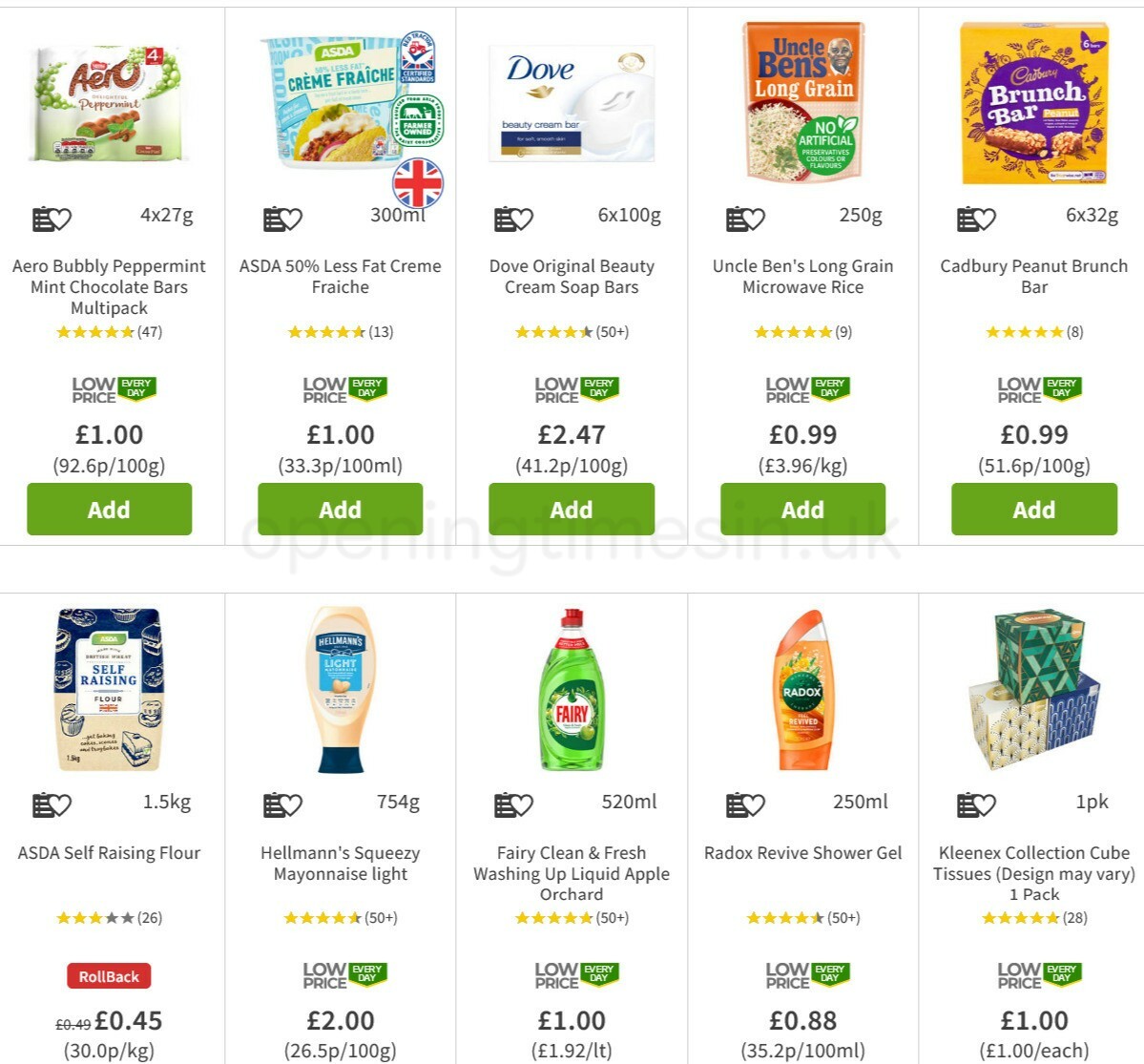**Caption:**

In this square-format, color screenshot, we see an online food and goods purchasing website featuring multiple well-known products. Although the specific site isn’t clearly identified, the branding indicates it is an Asda website. Prominent product listings include Aero Bubbly Peppermint Mint Chocolate Bars Multi-Pack, Asda brand Crème Fraîche, Dove Soap, Uncle Ben's Long Grain Rice, Cadbury Brunch Bar, Radox Shower Gel, and Fairy Washing Up Liquid, among others. Each item is accompanied by an "Add" button for easy selection.

Notably, the platform highlights "Low Price Every Day" for most products, and emphasizes special discounts with a "Roll Back" feature. One example is the Asda Self Raising Flour, originally priced at 49p, now reduced to 45p. Additionally, product ratings are visible, allowing customers to make informed decisions based on a five-star scale.